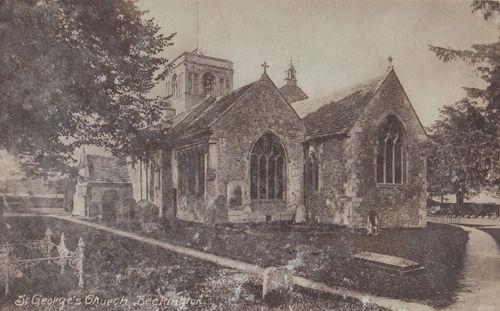This sepia-toned photograph, though damaged and of poor quality, captures the essence of St. George's Church in Beckington. The image features two side-by-side buildings with peaked roofs, each crowned with a prominent crucifix. These structures possess arched windows along their walls, adding to their classic architectural appeal. Surrounding the church, a yard extends to the front and side, with a large tree partially obscuring the left side, while another tree stands to the right, framing the scene. Despite its aged and somewhat ambiguous nature, the photograph's sepia tone gives it a distinguished, historic feel. In the lower left corner, the text "St. George's Church, Beckington" is faintly visible, identifying the old, storied church. Additionally, a small cemetery with a few tombstones can be seen on the left side of the image. The photograph provides a nostalgic glimpse into the past, showcasing the timeless exterior of this venerable church.